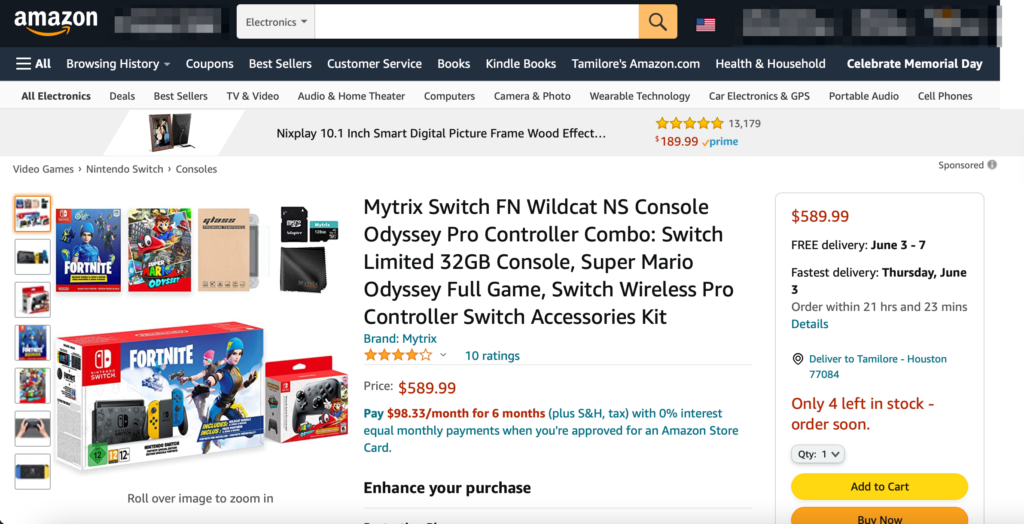This is an image of a horizontal web page screenshot displaying the Amazon website. The background of the page is white, and the Amazon logo is prominently positioned in the upper left corner. A search bar, accompanied by a search icon and a flag, occupies the upper top banner of the site. Below the top banner, a navigation bar featuring different categories sits on a dark grey background, followed by an electronics selection bar on a white background.

On a light grey banner situated beneath these elements, a featured product is highlighted: the "Nixplay 10.1 inch Smart Digital Picture Frame" with a wood-effect finish, boasting a 5-star rating and priced at $189.99. To the right of this product description is the main featured product, accompanied by several images and different views. The product is detailed as the "Mitrex Switch FN Wildcat NS Console, Odyssey Pro Controller Combo, Switch Limited 32GB Console, Super Mario Odyssey Full Game, Switch Wireless Pro Controller Switch Accessories Kit," by the brand Matrix. This item has received a 4-star rating and is priced at $589.99.

Below the product information is a section detailing payment options. To the right of the product details is a vertical box indicating shipping and stock information: "Free delivery June 3rd through 7th" and "Only 4 left in stock. Order soon." The box also features two prominent purchase buttons—a yellow "Add to Cart" button and an orange "Buy it Now" button. The rest of the information on the page has been blurred out, keeping the focus on the highlighted products.